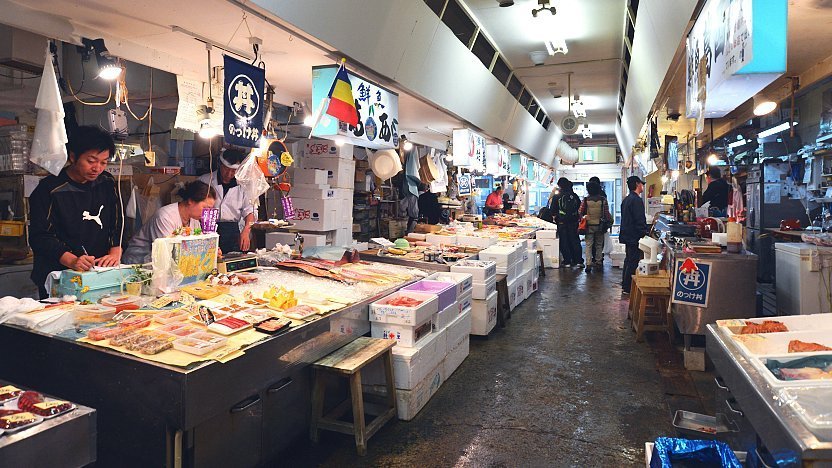The photograph captures a bustling scene inside an Asian market or food store, characterized by a long hallway lined with various vendors. The room is brightly lit by LED or fluorescent lights hanging from the ceiling, illuminating the colorful array of products on display. On the left side of the image, three focused vendors are working at a table, examining and possibly cataloging items, some of which include seafood and different types of meat housed in white styrofoam boxes. The tables are covered with vibrant, colorful objects, and flags and flyers with Asian script adorn the walls, emphasizing the cultural setting. There is a glass case near the front of the scene where a customer is interacting with a salesperson. Further down the aisle, additional people can be seen moving about, adding to the lively atmosphere of the market.Overall, the detailed elements highlight a typical day in a market within an Asian country, emphasizing the diverse array of products and the bustling activity of vendors and customers alike.